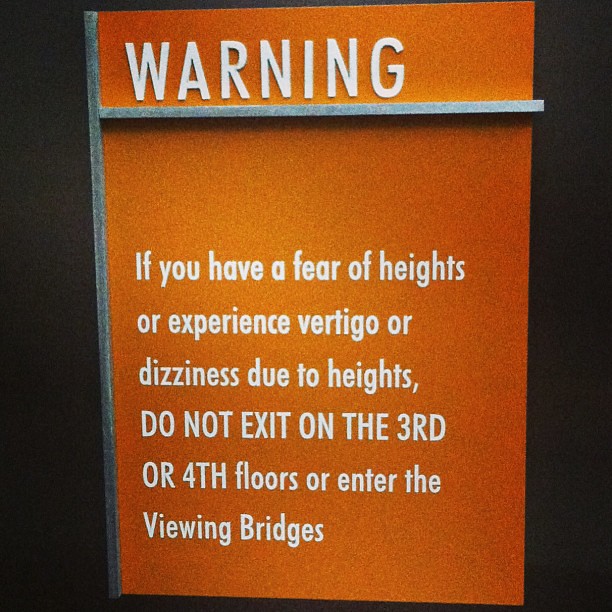The image depicts an orange sign with white text that prominently features a warning about vertigo and fear of heights. At the top of the sign, in larger white lettering, the word "WARNING" is displayed, underlined by a small gray bar. Below this, the sign cautions, "If you have a fear of heights or experience vertigo or dizziness due to heights, do not exit on the third or fourth floors or enter the viewing bridges." This warning is specifically aimed at individuals who might encounter problems with heights on these higher floors, likely in a high-rise building or a similar structure. The background of the image is predominantly black, and to the left of the sign, there is a steel barrier that extends partially into the image, adding to the structural context. The dimensions of the image are taller than it is wide, contributing to the overall framing of the warning sign.